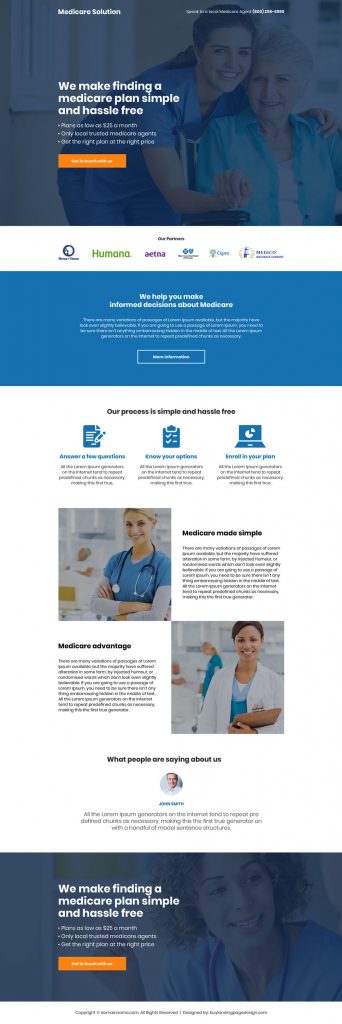The screen capture displays a web page with a clean, white background, featuring various images and text segmented by blue and gray rectangles. At the top, there's a prominent image of two women; one is seated on a chair while the other leans over her shoulder. Both women are dressed in blue attire. Superimposed on this image is white text that reads, "We make finding a Medicare plan simple and hassle-free."

Beneath this, several smaller images depict different professionals: a woman dressed in blue scrubs with long white sleeves, and another woman clad in a white lab coat, presumably a doctor. Below these images is a grayed-out photograph of a smiling woman, also overlaid with the phrase, "We make finding a Medicare plan simple and hassle-free." These elements collectively emphasize the site's focus on professional healthcare services, particularly in relation to Medicare plans.